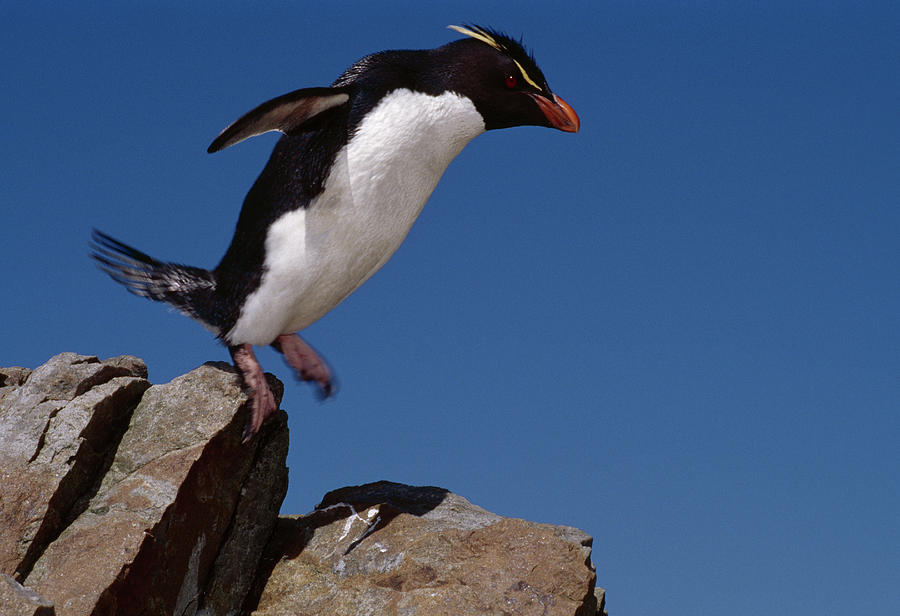The image captures an outdoor scene under a bright blue sky, showcasing three large, brown rocks. In the bottom left corner, a penguin is prominently featured, appearing to be in the middle of jumping or about to take flight from one of the rocks. The penguin, positioned near the center of the image, has a striking appearance with a white underside, black back, head, and neck. Its beak is vibrant orange, with a touch of yellow above its eye and ear. The penguin's feet are a dark orange-brown, and its tail is black. The color palette of the scene includes shades of blue, black, yellow, orange, tan, and gray, clearly indicating a natural, midday setting without any additional objects or text.